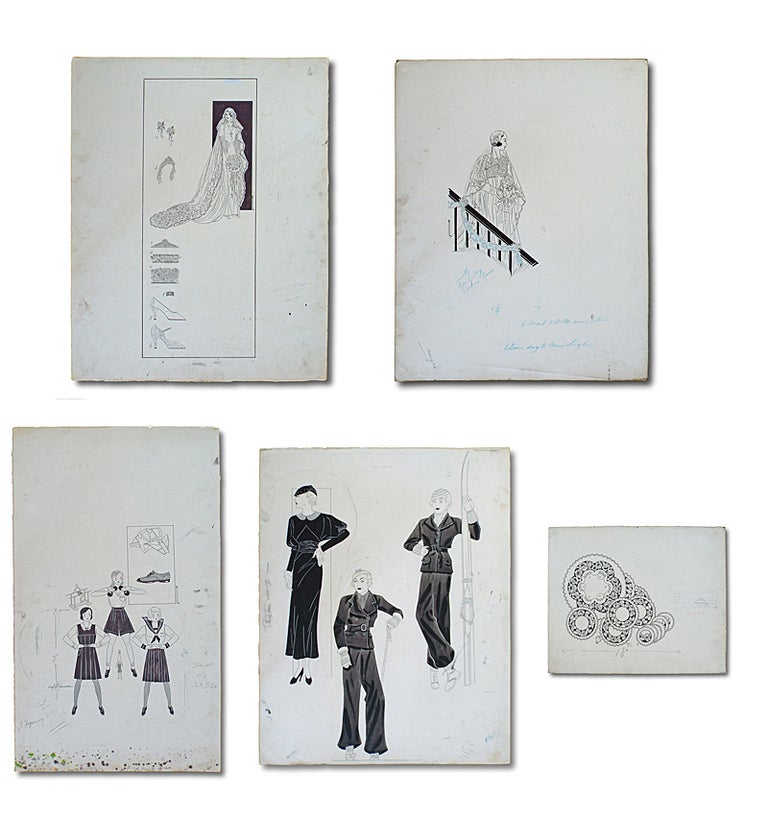This collection of vintage black and white illustrations, likely drawn with a darkened hue pencil, features five distinct hand-drawn images arranged in a square format, two on the top and three beneath. The top-left portrait depicts a woman in a wedding gown, holding a bouquet, framed against a rectangular black box with diagrams of high-heeled shoes. The adjacent top-right image shows another woman in bridal attire, adorned with a veil and headpiece, descending a dark, almost-black staircase banister. Both top illustrations are roughly 8 by 11 inches. 

Below, on the bottom-left, three women are captured in various athletic poses: one lifting weights and two with hands on their waists. This image displays weathering, evident by black and green speckles resembling mold, and includes sketches of folded uniforms and shoes at the top. The center bottom image showcases the same woman in multiple outfits: a black ankle-length dress with a white collar, a dark gray or black pantsuit with a white polka-dot hat, and another pantsuit while holding skis. The final, smallest image on the bottom-right presents intricate circular decorative patterns, reminiscent of plates. All illustrations exhibit a vintage 1950s-era aesthetic, evoking a sense of nostalgia and reflective of a bygone era.